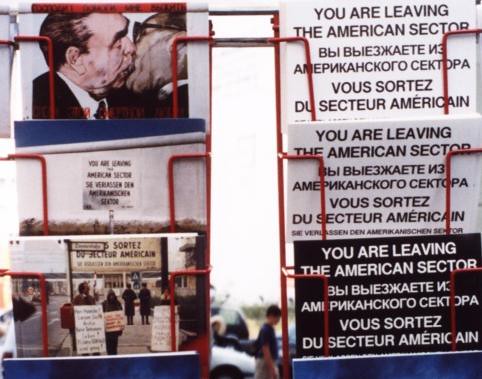The image features a smaller square format predominantly filled with blue and white hues. Centrally and along each side, there are red wire newspaper racks reminiscent of older outdoor stands. These racks contain various postcards or signs neatly arranged in two rows with three items each. Prominently, the top left slot showcases an image of two older men kissing. Below it, the middle slot holds a nondescript sign with blue and white elements, and the bottom slot displays people engaged in picketing with a partially readable sign mentioning "sortez something American."

On the right side, the top slot contains a postcard with a white background and black text stating, "You are leaving the American sector," accompanied by text in a foreign language. This message is repeated in the middle right slot, again on a white background. The bottom right slot features the same phrase but set against a black background. In the blurred background are indistinct people and partial views of vehicles under a sky-like expanse, adding depth to the vivid, detail-oriented composition.